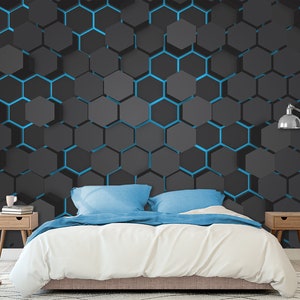This image is a 3D color illustration of a modern bedroom, created using a design app such as SketchUp. The focal point is a low profile bed, featuring a tan box frame and a thick, plush white comforter. Blue sheets, folded back, and blue pillow covers match the decorative accents in the room. The bed, potentially a full or queen size, is flanked by two nightstands. Each nightstand is a beige wood piece with a single drawer and four long, dowel legs. On the left nightstand, there are books and possibly a small mug, while the right one is bare.

Behind the bed, most of the wall is adorned with a dark gray honeycomb (or beehive) pattern adorned with light blue accents along the edges of some hexagons, adding a cohesive touch to the bedding. Adding a modern touch, a silver lantern light is mounted on the right side of the wall, partially cut off in the image. The bed's width spans across the entire bottom of the image, emphasizing the cozy and detailed interior design.